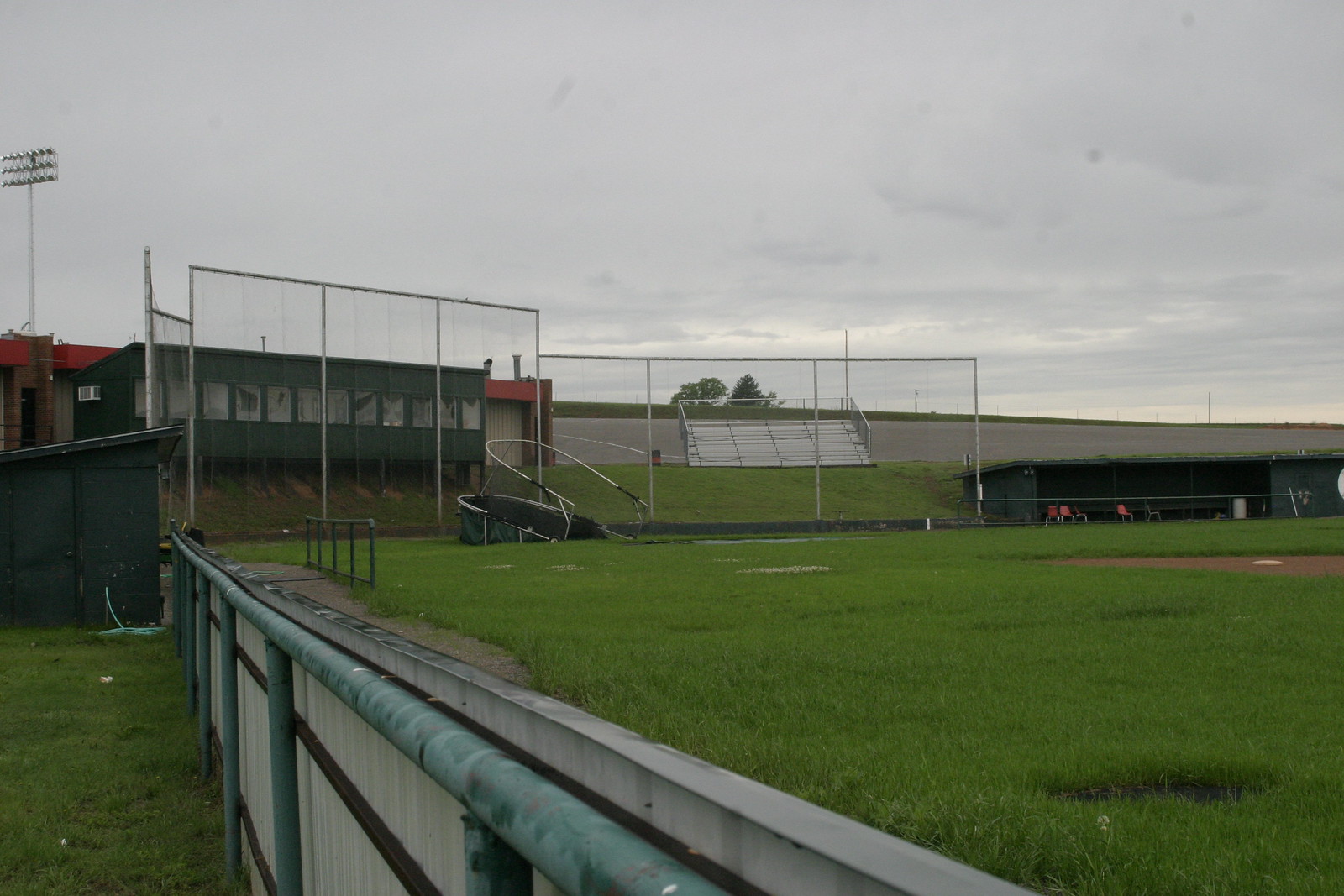The image captures a baseball field with vivid green grass and a distinct diamond including home plate and the pitcher's mound, although it appears not ready for use. There's a low white and metal fence surrounding the field, transitioning to a taller chain-link fence that shields potential spectators in the stands from stray balls. Two green dugouts are visible on either side of the field; one contains red chairs. A green press box with windows sits behind home plate, beneath which are unoccupied seats. The sky overhead is gray and cloudy, bordering on dark, casting a moody ambience over the scene, which is devoid of any players or fans. Beyond the stadium's fence, trees frame the setting, suggesting it might be early spring or late fall.